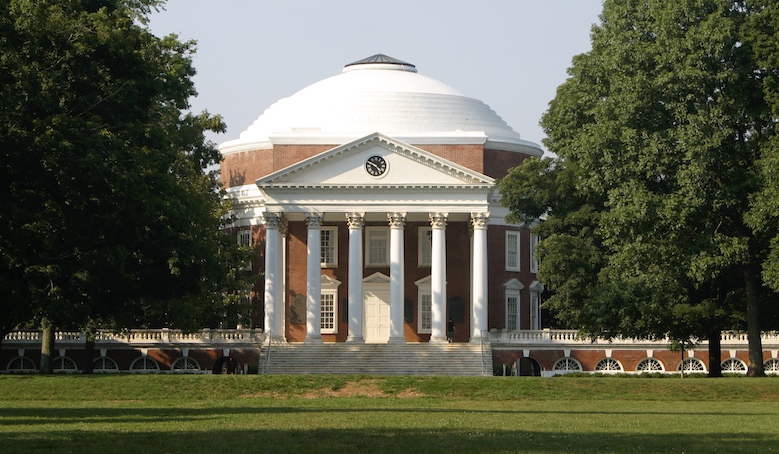The image captures an outdoor scene on a sunny day, taken from a green lawn with patches of brown dirt. The focal point is a white-domed building with a circular skylight at the top. The dome is supported by six white columns under a portico with a peaked roof featuring a clock. The building's exterior walls are a dark brown or dark orange brick, complemented by white windows and a door. Flanking the building are two large trees with dark green leaves, positioned on the left and right sides of the photograph. The clear blue sky provides a vibrant backdrop to this horizontal, rectangular image.